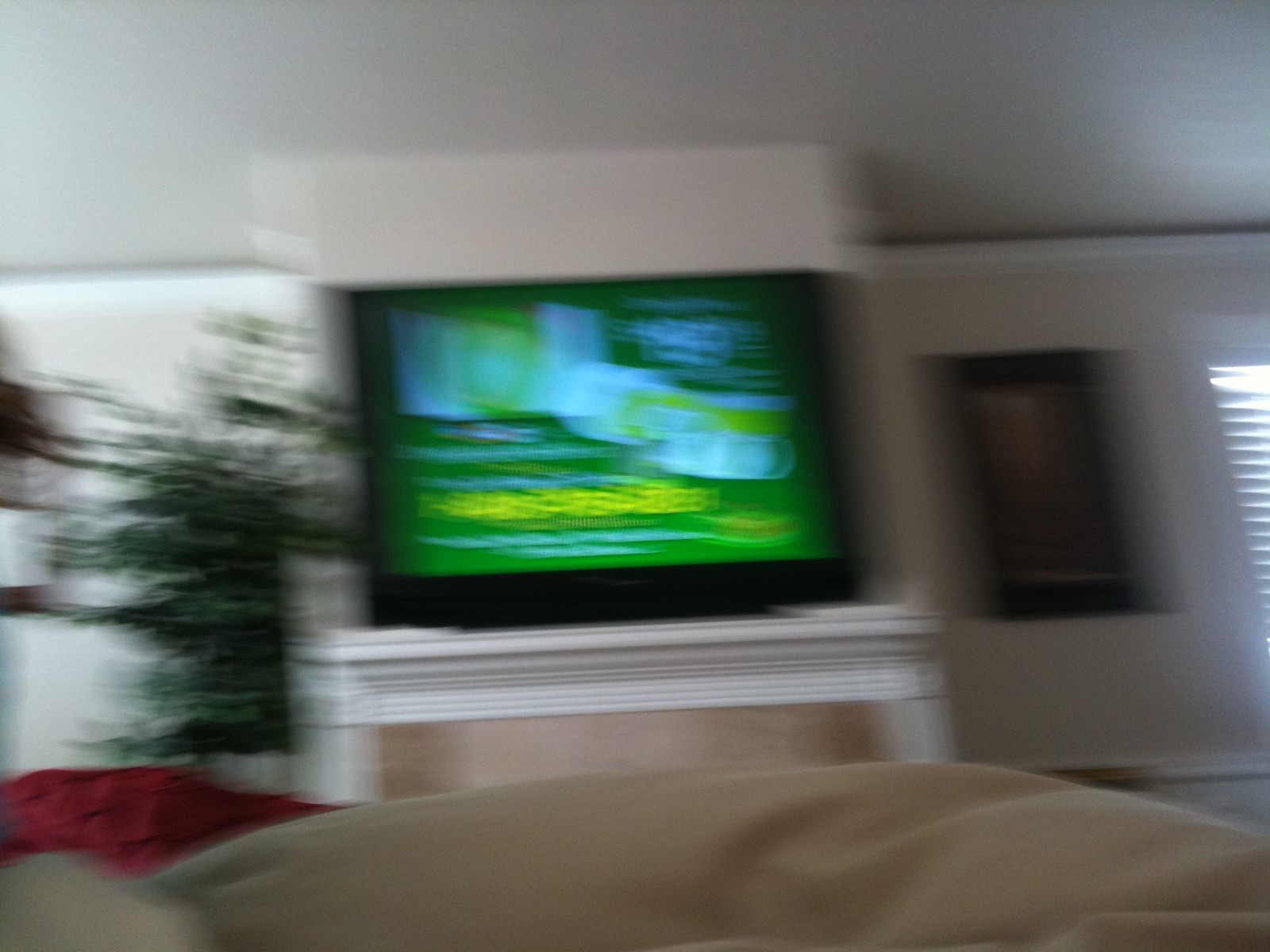This photograph, taken from the perspective of someone seated on a couch in a living room, is characterized by significant blurriness due to the camera being in motion. Central to the image is a TV screen, mounted on a wall above what appears to be a fireplace, though the exact details are indistinct. To the left of the television, there is a hanging plant in a pot or shelf, adding a touch of greenery to the space. To the right, a vertically framed painting or photograph is visible, but its content is obscured by the blur. The TV screen itself displays an advertisement featuring prominent colors of green, yellow, and white, although the precise details remain unclear due to the motion-induced blur.